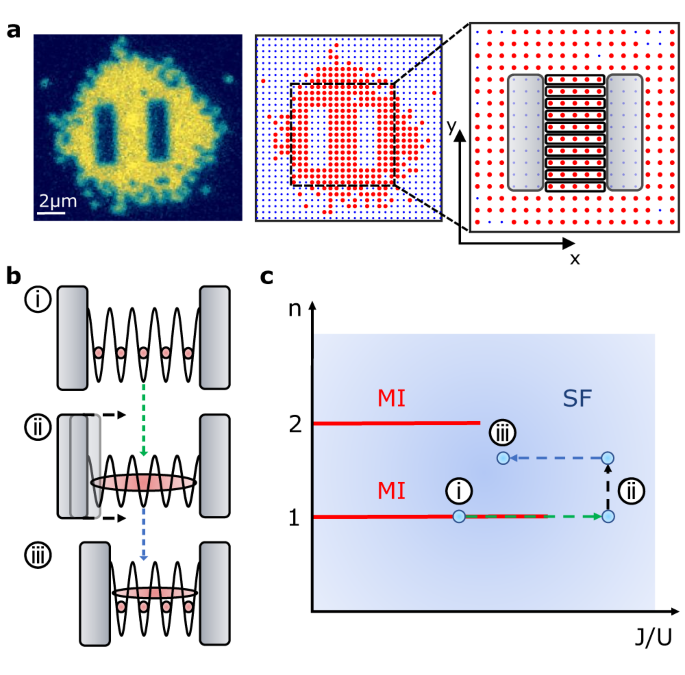The image displays three complex scientific diagrams, labeled A, B, and C, set against a white background. Diagram A consists of three sequential frames. The first frame features a blue background with a yellow microorganism-like shape at the center, encased by a blue irregular outline. Within this shape are two vertical blue rectangles. The second frame transitions to a grid filled with predominantly red dots, except for two vertical areas of blue dots. The final frame in Diagram A shows an X-Y coordinate system, with red-dotted surroundings and two vertical silver rectangles, flanked by horizontal red rectangles.

Diagram B is composed of three vertical illustrations depicting energy transfer between two gray piers. These illustrations resemble an accordion-like structure with squiggly lines and red ovals representing varied stages of energy flow.

Diagram C, the final one, presents a chart with an N labeled on the top and JU on the bottom, plotting two lines marked 1 and 2. Both lines are red, with one line extending to include three dotted projections beyond the main red line. 

Overall, these diagrams appear to have detailed scientific notations and symbols such as MI and SF, commonly used in fields like physics or chemistry. However, the absence of explanatory text makes it challenging to determine their exact significance or application.